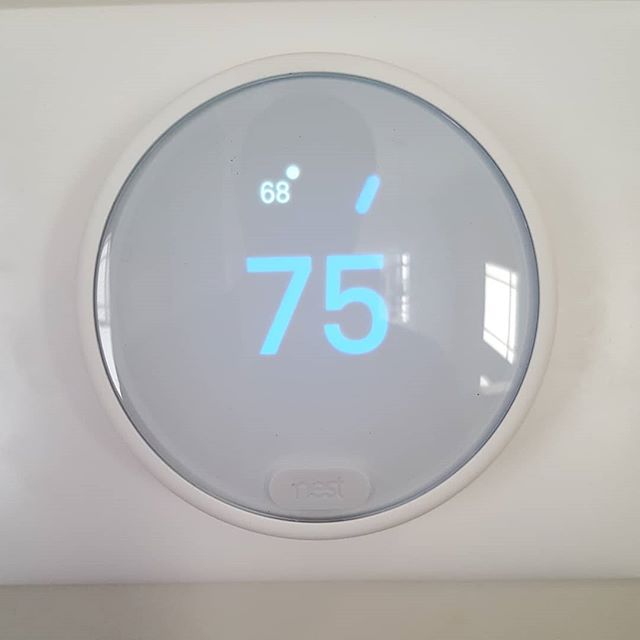A close-up image of a white wall-mounted thermostat for an air conditioning unit, featuring a digital readout. The thermostat has a round digital window with a gray background, encased in a white frame. The main display shows the current temperature in large, blue numerals: 75 degrees Fahrenheit. Below, a smaller white number indicates the set temperature: 68 degrees Fahrenheit. Covering the digital window is a translucent plastic dome. At the bottom of this dome, there is a lozenge-shaped brand name tag, which appears to be embossed with "Nest," making it slightly challenging to read.